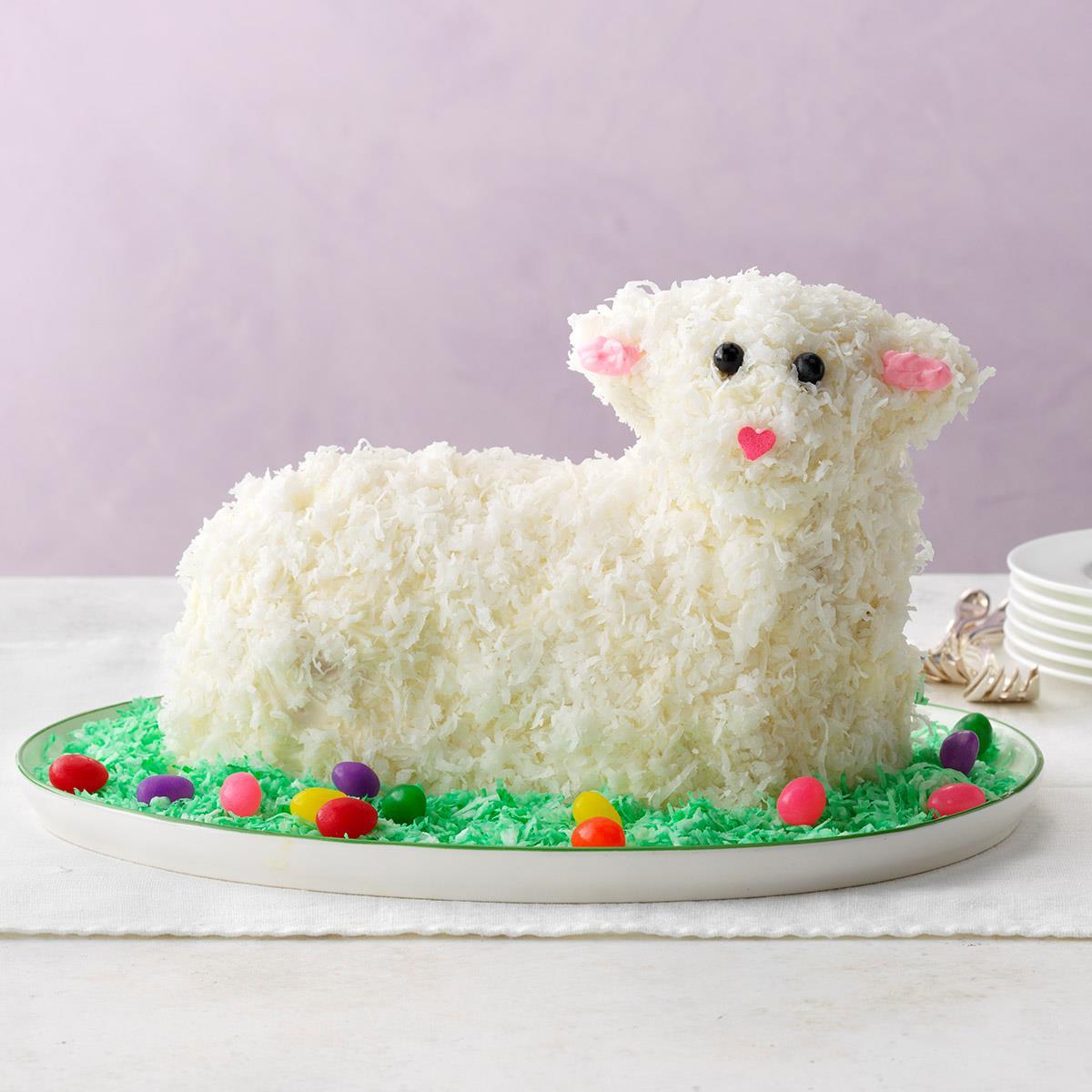In this vibrant and charming image, we see an intricately decorated lamb cake, meticulously crafted to appear fluffy with a generous coating of white coconut icing, adding a textured, wool-like effect. The lamb's eyes are two black jelly beans, giving it an adorably beady look, and its nose is a cute pink heart made of icing. The ears are highlighted with pink icing as well, enhancing its endearing appearance. The cake is artfully placed on a bed of bright green icing designed to look like Easter grass, with an array of colorful jelly beans—bright pink, purple, green, yellow, and red—scattered across the platter, creating a festive atmosphere. In the background, the scene is framed by a purple backdrop, a white tablecloth, and visible are two silver forks and five white serving plates, potentially ready for a delightful tasting.